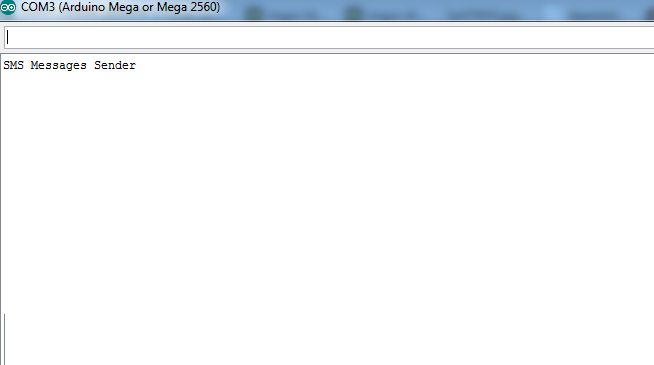Screenshot of a Display Interface with SMS Functionality

The screenshot captures a display interface featuring a dark blue banner at the top. This banner contains a circle icon with plus and minus signs, followed by the label "COM3" and "Arduino Mega or Mega 2560" in parentheses, indicating the communication port of an Arduino device.

Beneath the banner, there is a white rectangular input box with a blinking cursor, suggesting it is ready for text entry. Below this input field, the screen extends into a larger white background area framed by a black bar at the top and along the left side.

Centered within this white background area, there is a black-text label that reads "SMS MESSAGES SENDER" in capital letters. No SMS messages are displayed, indicating that the screen currently has no messages or senders listed. The interface appears to be awaiting input or further interaction to display sent or received SMS messages.